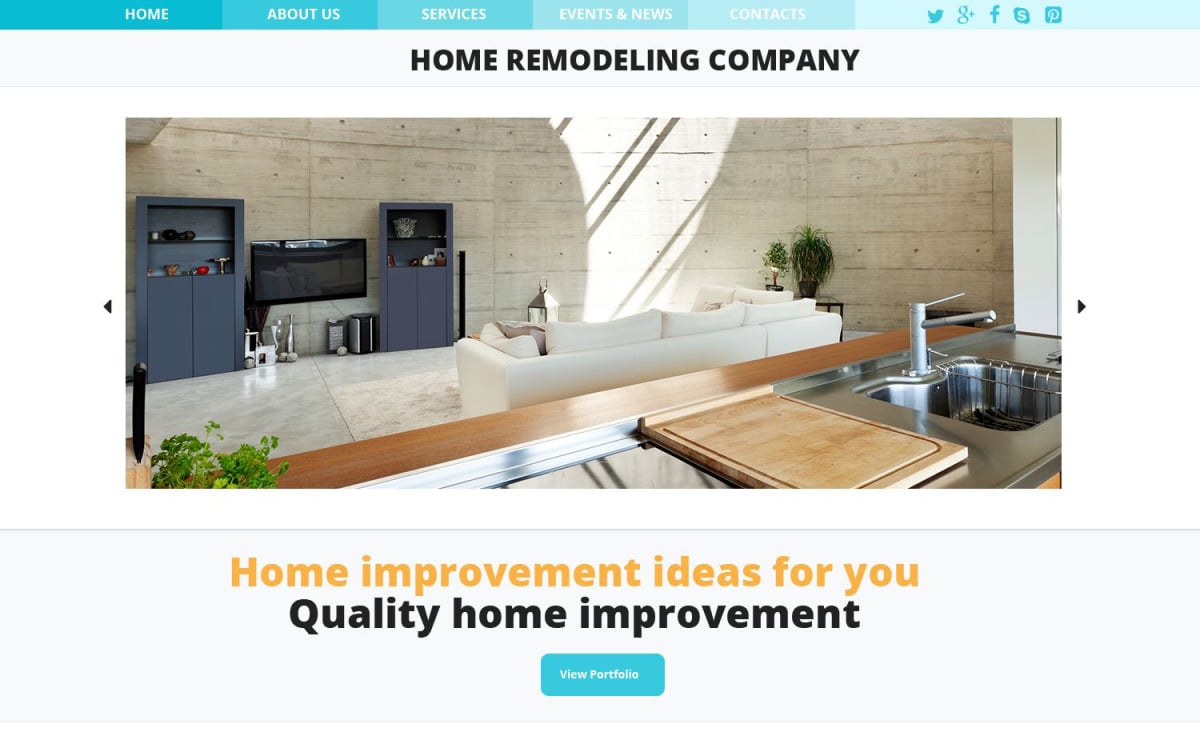This image, captured from a home remodeling company's website, showcases a stunningly remodeled living space. The focal point is a cozy living room featuring wall-mounted shelves. To the lower right, a glimpse of the adjacent kitchen reveals a sink and cutting board. Soft natural light filters through, casting delicate shadows on the background walls, adding to the room's inviting atmosphere.

The website's navigation bar is highlighted by a gradient teal strip at the top. The gradient transitions from dark to light teal as it extends from left to right. The bar includes menu options labeled "Home," "About Us," "Services," "Events and News," and "Contacts." Social media icons for Twitter, Google+, Facebook, an 'S' (possibly for Snapchat or another service), and Pinterest are also prominently displayed.

At the bottom of the page, a gray rectangular banner contains the tagline "Home Improvement Ideas for You" in eye-catching yellow print. Below this, black text reads "Home Improvement," and the final line features a teal-colored box with the call-to-action "View Portfolio." The concise, clean layout effectively combines aesthetic appeal with user-friendly navigation, reflecting the company's professional image and dedication to home improvement.